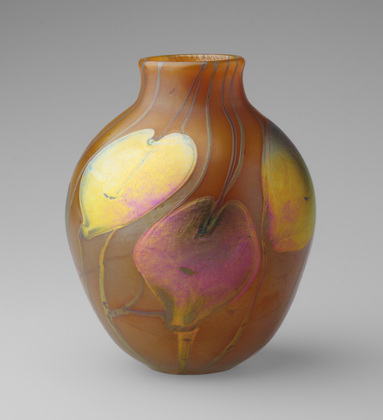The image depicts a photograph of a circular vase with a large base and a smaller top opening, set against a plain, light gray background. The vase is made of a material that resembles glass, featuring a dark amber or brownish-orange color. Adorning the vase are three heart-shaped or lily pad-like decorations: one on the left in bright yellow, one in the center in a pinkish-red hue, and one on the right that is a mixed shade of yellow and pink. These shapes have beige stems and are accompanied by swirling lines in gray as well as thin, blue lines that extend from the top downwards. The overall aesthetic is simple yet detailed, combining shapes and colors with an elegant, flowing design.